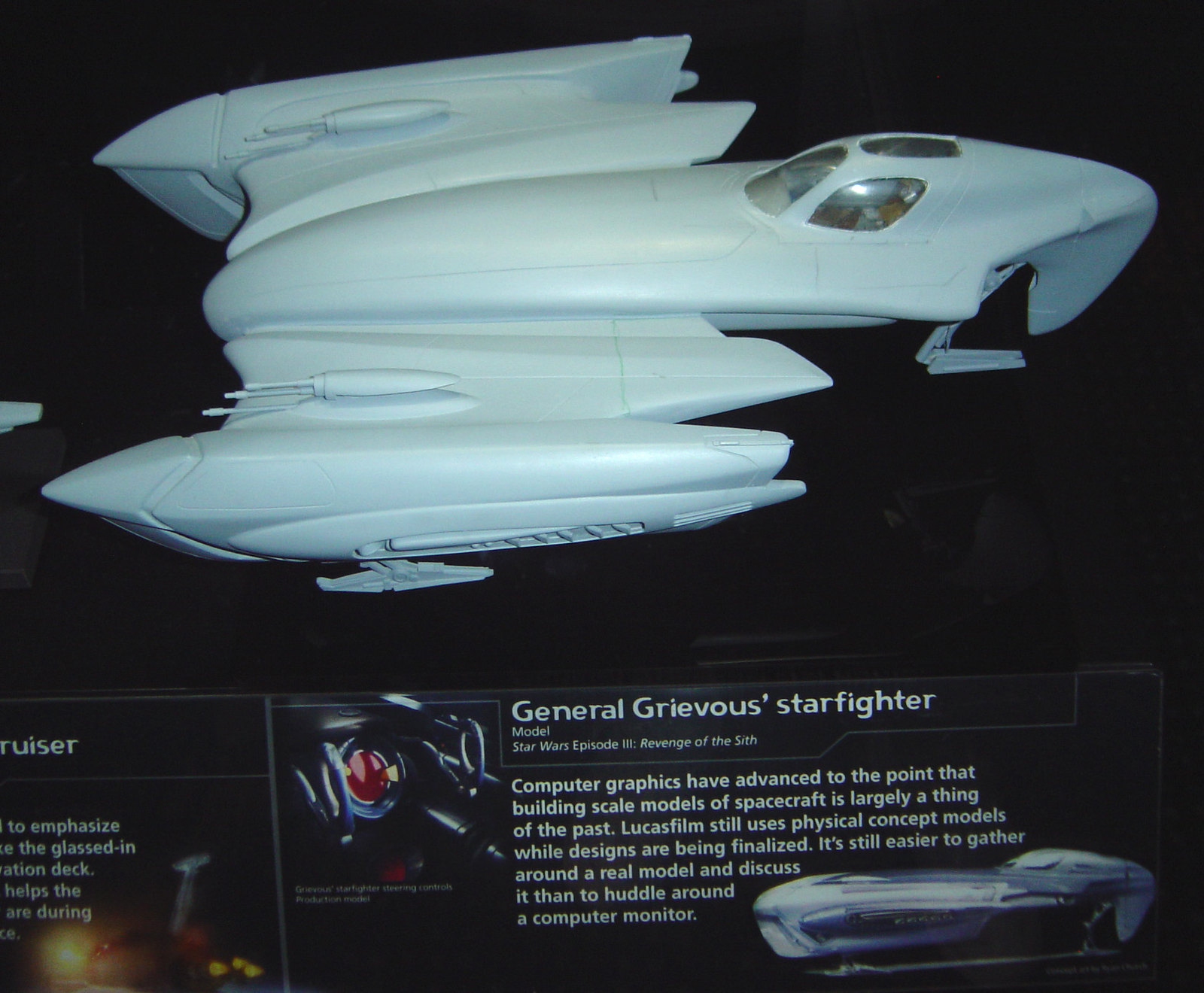The image is a horizontal rectangular photograph or computer-generated rendering depicting a futuristic aircraft, likely a conceptual design or a model from a movie. The top portion showcases the sleek and advanced design of the General Grievous Starfighter from Star Wars Episode 3: Revenge of the Sith. The aircraft features noticeable guns and windows, though its unconventional shape is challenging to describe in detail. The background is predominantly black, emphasizing the starfighter's form. 

Text appears at the bottom of the image in white font, mentioning details about the computer graphics and the design process. The primary caption, close to the center but slightly right-aligned, reads "General Grievous Starfighter Model Star Wars Episode 3 Revenge of the Sith," with additional smaller, less legible text explaining the evolution of spacecraft modeling. Notably, it mentions how Lucasfilm still uses physical models during the design stages because they facilitate more effective collaboration compared to digital models.

Within the image, there's a close-up of the starfighter's interior on the lower left, showing a detailed view of the pilot's central control area, potentially the steering mechanism. Another red-circled inset image on the right-hand side gives an additional perspective of the starcraft. The left side of the image also contains cut-off information, suggesting there might be more text or details that are not fully visible.

Overall, the image highlights the hybrid use of physical and digital modeling in modern spacecraft design, with a focus on the iconic General Grievous Starfighter from the Star Wars saga.